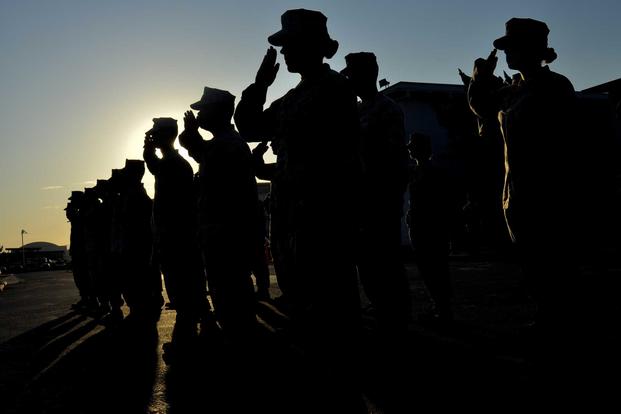In this dramatic image taken at either sunrise or sunset, a line of approximately ten soldiers stands at attention, their hands raised in salute. The soldiers are silhouetted against the fading light, rendering them as dark shapes, which adds to the solemn atmosphere. The diverse group includes both men, identifiable by their short hair, and women, discernible by their buns or ponytails. They stand on what appears to be concrete ground, likely at a military base, with clear skies overhead. In the distance, various vague structures can be seen, including a square building and what looks like a tent. The sun is positioned directly behind the soldiers, casting their features into shadow and making individual details indistinct, save for their distinct ceremonial posture and military hats.